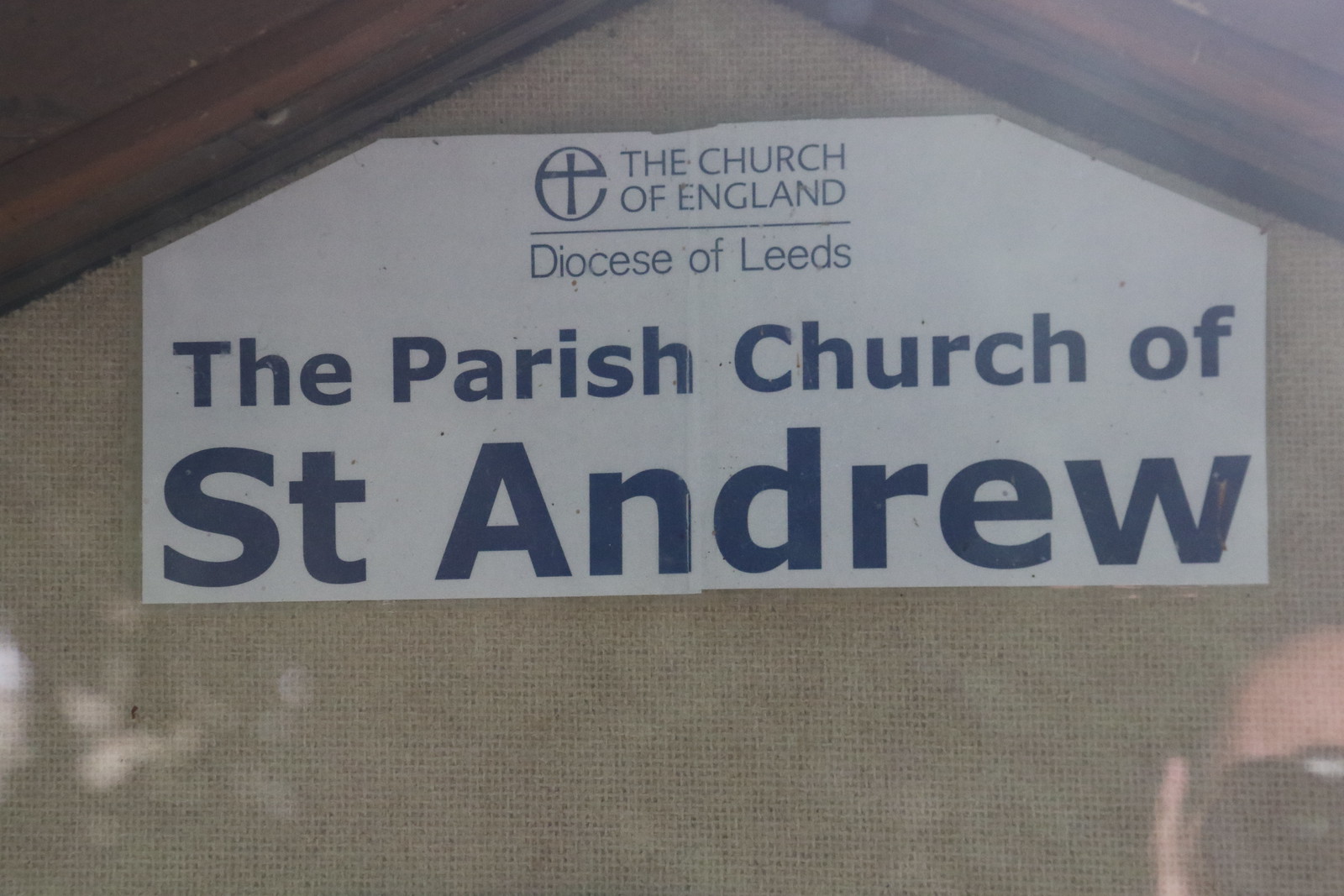This image depicts a detailed view of a signage banner positioned within a wooden frame resembling the peak of a church roof, likely framed with brown wood and set against a beige or cream-colored background. The scene appears to be outdoors, suggested by the reflection of a person with short hair wearing sunglasses in the glass case covering the sign. The upper portion of the banner features a blue cross within a round, slightly imperfect circle, forming the letter "E" and displaying the text "The Church of England" in blue print. Below it, separated by a divider line, the words "Diocese of Leeds" in bold black letters stand out. The bottom portion prominently declares in progressively larger text, "The Parish Church of St. Andrew." The elements suggest that the banner might consist of two sheets joined together to ensure the text's visibility. The image was taken during daylight, evident from the brightness illuminating the scene.